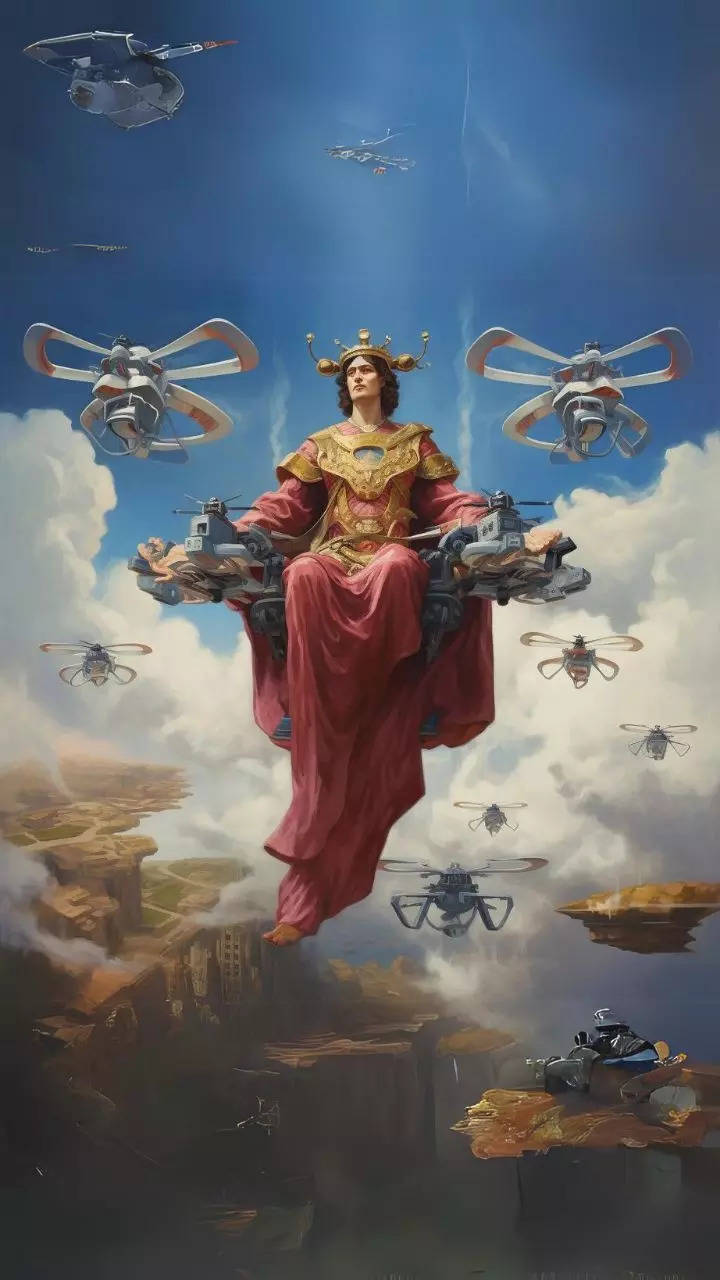The image appears to be a painting or an AI-generated graphic of a majestic figure seated on a high-tech, floating throne. This supernatural visual presents a person, donned in a long red robe or cape and adorned with a golden crown and chest plate, suspended in the sky with a backdrop of blue sky and white clouds. Surrounding the figure are numerous butterfly-like drones or UFOs with rotors and wings, colored primarily grey with red accents. Beneath this celestial procession, a varied landscape unfolds with glimpses of land, mountains, and possibly the remnants of a city amidst greenery. The scene blends realistic and fantastical elements, depicting an ethereal ascent from the earthly domain below to the expansive heavens above.